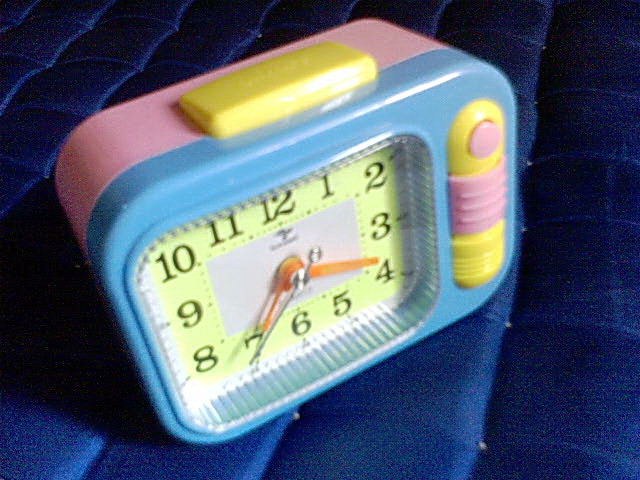The photograph showcases a small, rectangular toy alarm clock designed for young children. The clock is placed on a dark blue bedspread with a quilted pattern. The vibrant aesthetic features a light blue front with a pink back, and additional colorful components that make it visually appealing to kids. The top of the clock has a raised rectangular yellow button in the center, likely meant for setting or stopping the alarm. Positioned on the right side of the front, there is a vertical yellow section with a spherical pink button on top and a central square with ridged lines, hinting at an interactive element that children can slide.

The clock face, situated on the left side, is encased in clear plastic. It has a yellowish-green background with bold black numbers from 1 to 12, making it easy for children to read. The hands for the minutes and hours are orange, while the second hand is a thin, silver needle. The time displayed appears to be around 7:24. Overall, the clock's design is not only functional but also engaging for its young audience with its bright, playful colors and user-friendly buttons.